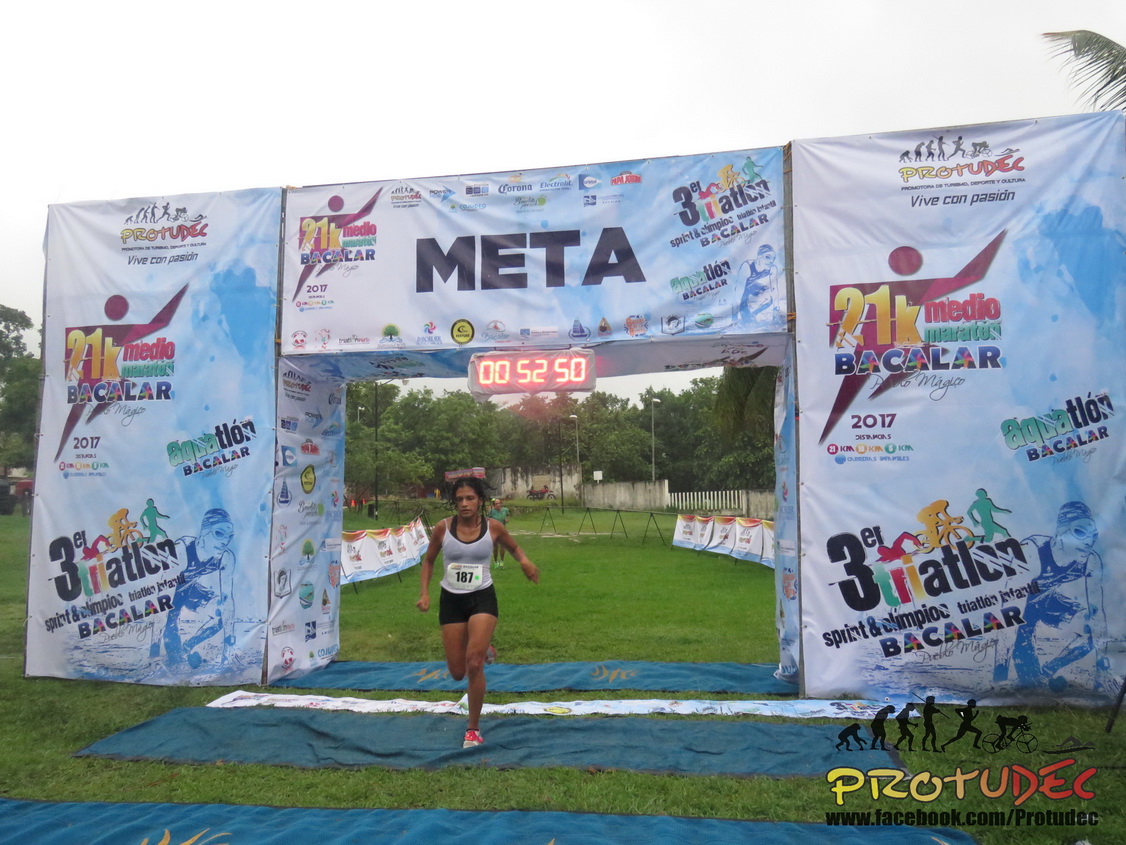The photograph captures the triumphant moment of a woman completing a race, crossing the finish line under a large rectangular structure marked with the word "META" in black letters at the top. The structure consists of two vertical, three-dimensional towers on either side, connected by a horizontal banner. Above the finish line, a digital timer displays "00:52:50" in red. The woman, who has dark hair, is dressed in a white tank top with a bit of black fabric visible underneath, black shorts that reach her upper thighs, and red sneakers with pink laces. She is also wearing a race number, "187," pinned to her chest.

The setting is outdoors with green grassy ground and a backdrop of trees. Blue tarps or flooring material are spread out along the raceway, especially noticeable around the finish line. In the bottom right corner of the image, there's an evolution-themed graphic depicting a sequence from an ape to a human, culminating in a person on a bicycle. Below this illustration, the text "PROTUDEC" appears in yellow and red letters, and further below, the URL "www.facebook.com/progedec" is printed in black. The race event details are scattered across the structure, mentioning "21K Medeo," "Triathlon," and possibly other phrases that are partially obscured or in another language.